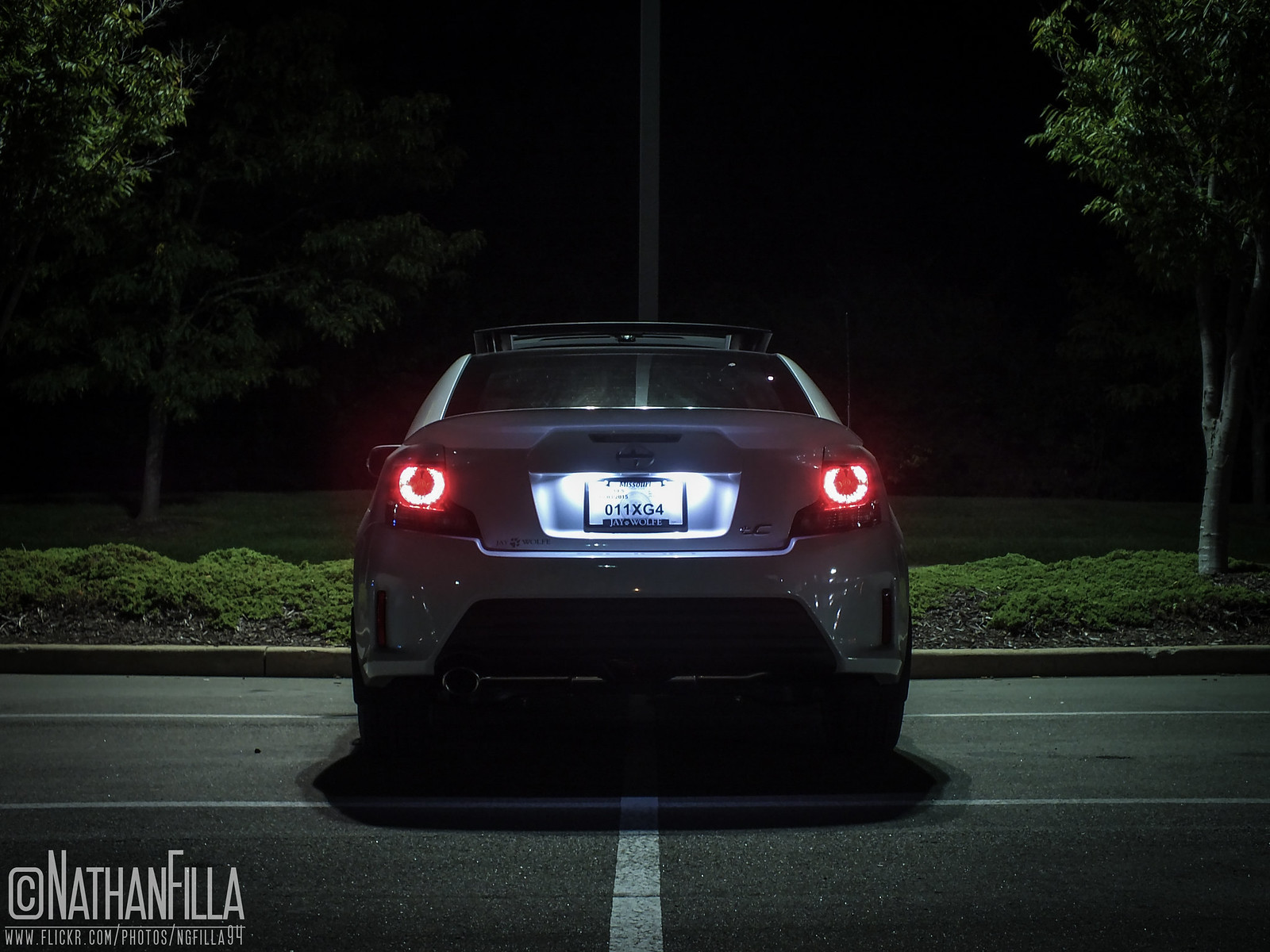This high-quality nighttime photograph captures a light-colored Scion, likely white or gray, parked in an empty parking lot beneath a streetlamp. Viewed from the rear, the car is positioned perpendicular to the parking spaces, creating a symmetrical and visually striking composition. The reflective paint gleams under the streetlamp, highlighting the car's well-maintained and possibly modified appearance, suggesting that the owner has invested in its upkeep. The car's circular red brake lights are illuminated, and its sunroof is open. The license plate reads "011XG4," with a distinctive backlit light nearby. The headlights are also on, subtly lighting the distance. Surrounding the car, trees and patches of grass are visible, enhancing the outdoor ambiance. At the bottom left, a watermark reads “Nathan Fila,” accompanied by the photographer's website, www.flickr.com/photos/ngfila94, emphasizing the image's ownership and professional quality.